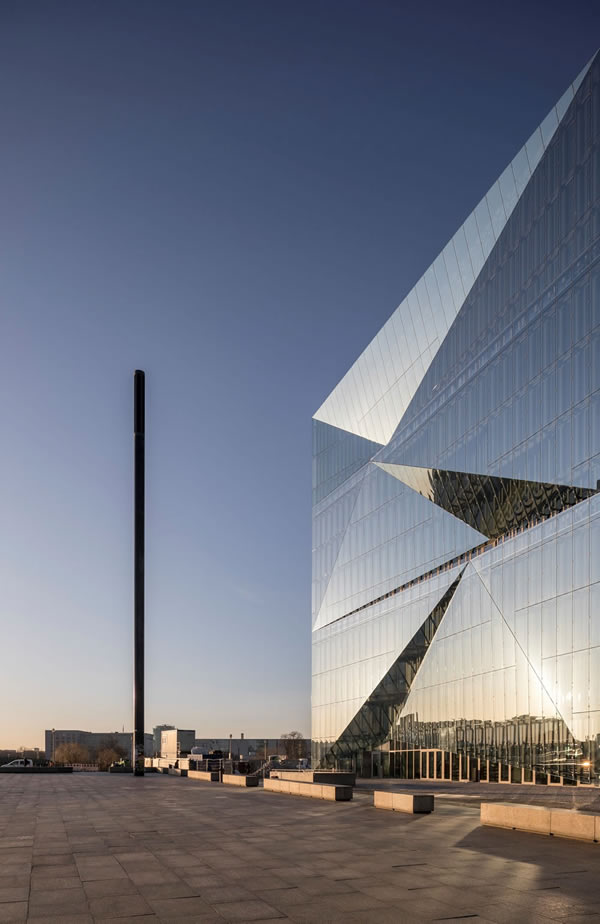This image captures an outdoor scene at either sunrise or sunset, with a dramatic, dark sky transitioning to blue with shades of yellow near the horizon. To the right stands a uniquely designed building composed of reflective glass triangles, resembling a crystalline structure. The building reflects the low sun, indicating it is either about to rise or nearly set. Spanning several stories, the building's angular, multi-faceted appearance gleams under the ambient light.

Prominently, a black flagpole without any flag stands to the left of the building, firm and noticeable. In front of the architectural marvel lies a meticulously laid walkway made of snugly fitting, dark grayish-brown square tiles. This area is furnished with plain, square or rectangular stone benches arranged methodically, serving as a seating arrangement.

In the far distance, a more traditional, rectangular building constructed of stone or concrete adds depth to the scene. Additional elements such as cars can be seen scattered in the background, subtly framing the foreground's tranquil and meticulously designed space.